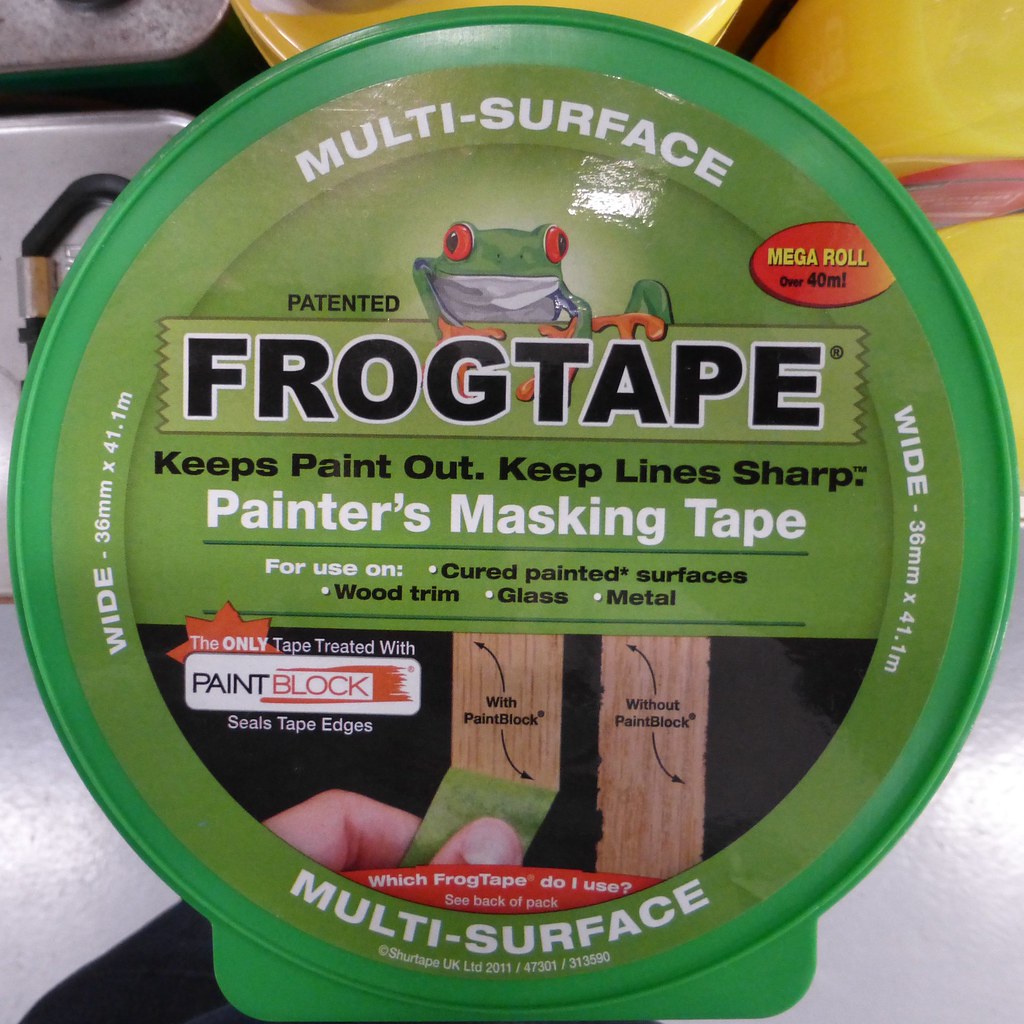This is a detailed photograph of the top of a circular green roll of Frog Tape, specifically a multi-surface painter's masking tape. The central label prominently features a green frog illustration with red eyes and orange feet and chin, climbing alongside the black text "Frog Tape." Above the frog, in an arch at the top, it reads "Multi-Surface" in white text. To the right of the frog, in yellow text on a red background, it states "Mega Roll," with "Over 40 meters" highlighted in black text beneath. Below "Frog Tape," additional black text reads "Keeps Paint Out, Keeps Lines Sharp," followed by "Painter's Masking Tape" in white text.

Further down, more detailed usage information is provided in white and black text: "For use on cured painted surfaces, wood trim, glass, and metal." There is also a comparison image illustrating the effectiveness of the tape with and without paint block technology, showcasing how the tape keeps paint lines sharp. A red note at the bottom advises, "Which Frog Tape do I use? See back of pack." Along the bottom arch and sides, the text "Multi-Surface" is repeated, and the dimensions of the tape are listed as "Wide 36 mm x 41.1 mm."

The background behind the tape shows colors of yellow, silver, and white, with additional materials and a person using the tape, demonstrating its application on various surfaces.